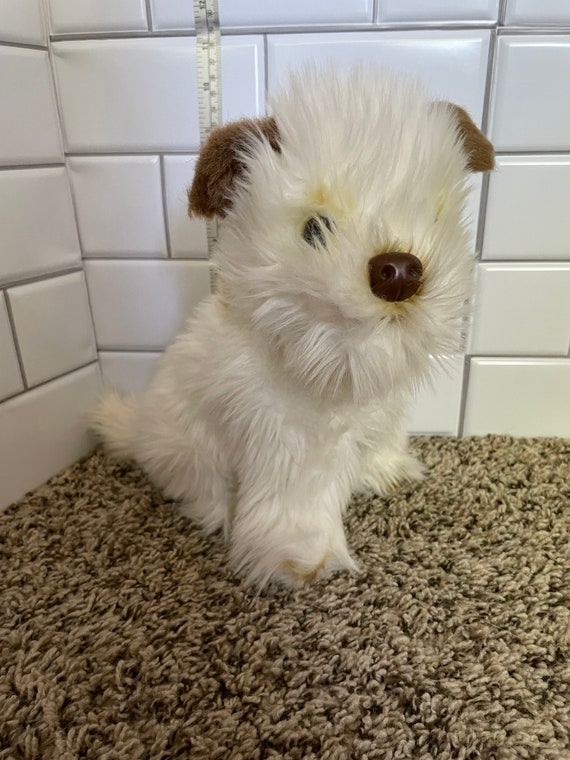This is a detailed photograph of a small, plush toy resembling a white dog, possibly a Pomeranian mix. The dog has soft, white fur with medium brown ears and a brown nose. Its eyes are dark, though only the right eye is fully visible as the fur partially covers the left eye. The toy is seated in the corner of a room on a brown, beige, and tan speckled carpet. The dog's tail touches the corner where two white, unevenly sized tiled walls meet at an obtuse angle, appearing more than 90 degrees. Directly behind the right ear of the toy is a white tape measure hanging down for scale, indicating the dog's height is approximately 9 inches. The dog is slightly angled to the right, with its front paws spread apart, giving it a lifelike appearance as it gazes toward the camera, creating a soft and inviting image.